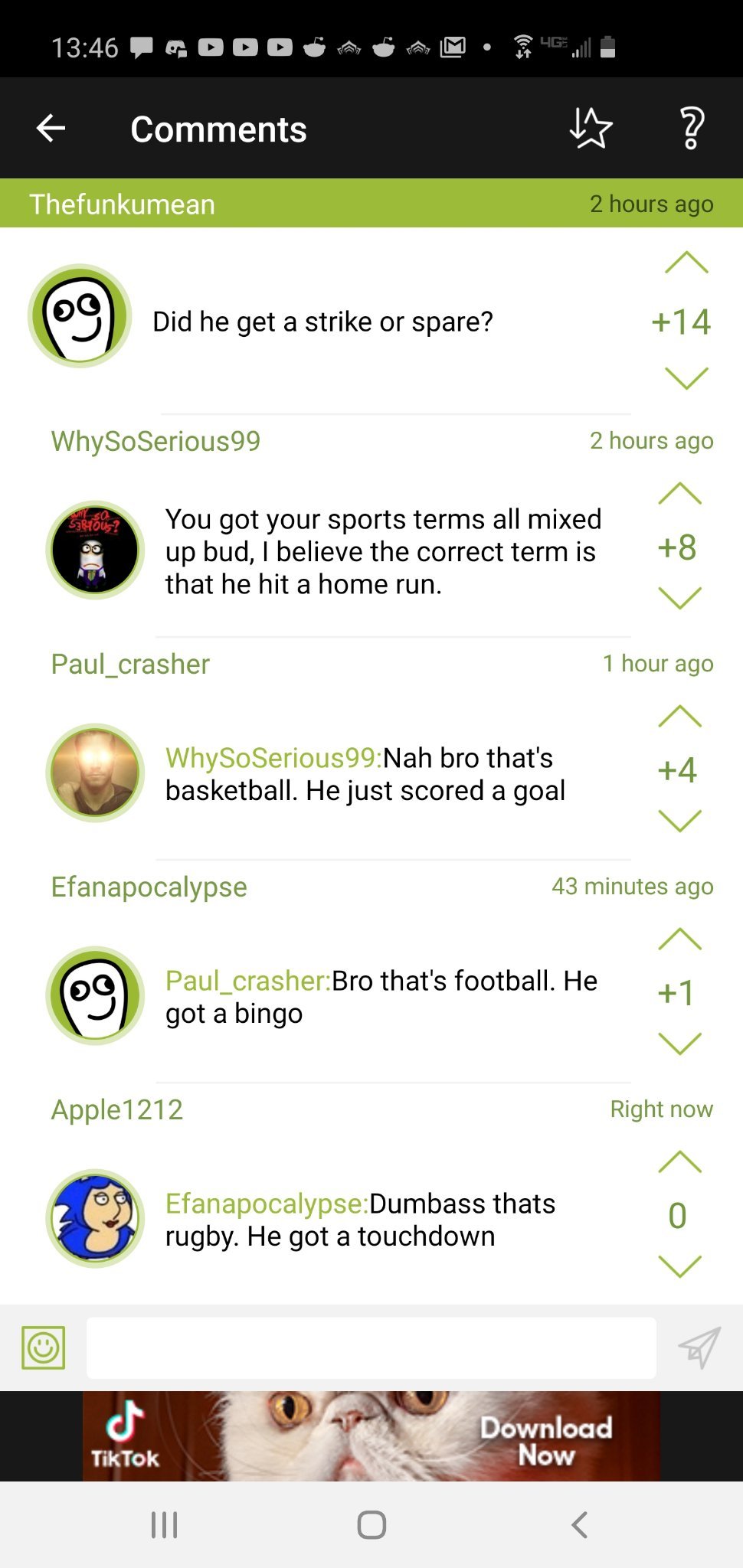The screenshot captures a portion of a smartphone screen displaying a Reddit comments section. At the top, a black background occupies the upper two inches. The top left corner displays "1346" next to various icons, including a message icon, three play icons, a Reddit icon, and another unidentified icon. Additionally, there are indicators for Gmail, Wi-Fi, 4G connectivity, and a half-full battery next to the time "13:46".

On the left side beneath the time, a bold white arrow points left, labeled "comments." On the right side, there's a bold, outlined question mark with a black interior and white border next to a star icon with a downward-pointing arrow on its left side. Below, a thin lime green border frames text on the left that reads "thefunkyoumean" in white, and on the right, "two hours ago" in black.

Below this section, the screen transitions to a white background extending down to about an inch from the bottom. Five comment threads are listed, each separated by a gray border. Each comment features a profile photo on the left, followed by the text of the message in the center, and upvote and downvote arrows on the right with numerical values in between. Notably, comments one and four are from the same user, while the others are from different users.

At the very bottom, a search bar is present, and below it is a black square with a TikTok advertisement. The ad displays a cat's face with text on the left reading "TikTok" and on the right, "Download now," showing only the eyes and the sides of the cheeks of the cat.

This detailed caption captures the intricate elements visible in the screenshot described.